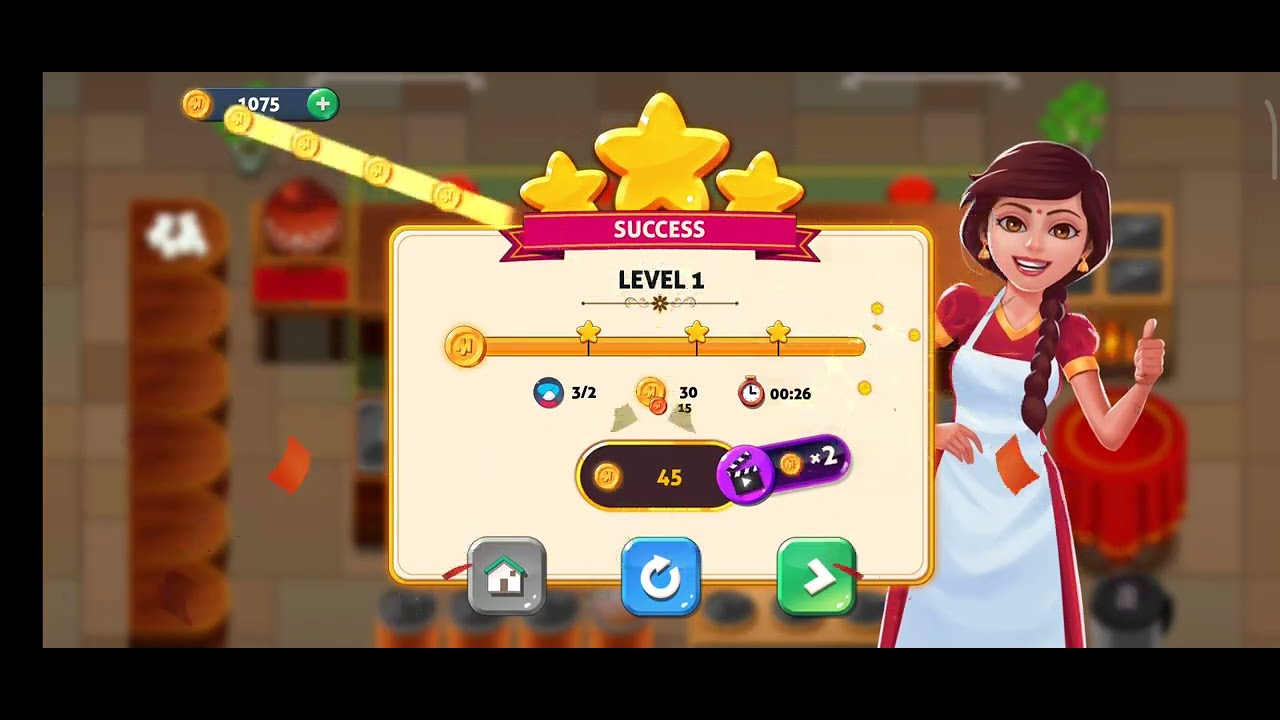This detailed caption combines elements from all three captions, emphasizing shared and repeated details:

This image is a screenshot of a video game, possibly an app for a cell phone. On the right side, there's a cartoon-style woman with brown hair in a long braid draped over her left shoulder. She is wearing a red dress, a white apron, and golden earrings. She holds her left thumb up, and has a dot on her forehead, indicative of a bindi. Part of her right side is obscured by a rectangular interface element. At the top of this rectangle, a ribbon bearing the word "Success" leads into the text "Level 1," with three horizontal yellow stars beneath it. Below the stars are some scores and additional icons; a house icon on the left, a replay symbol in the center, and a rightward-pointing arrow on the right. The background is blurry but suggests a game environment featuring a dining table, some tables, a window, and an orb. There are elements like a giant yellow line with stars extending from the left side upwards, adding to the overall celebratory theme of the scene.